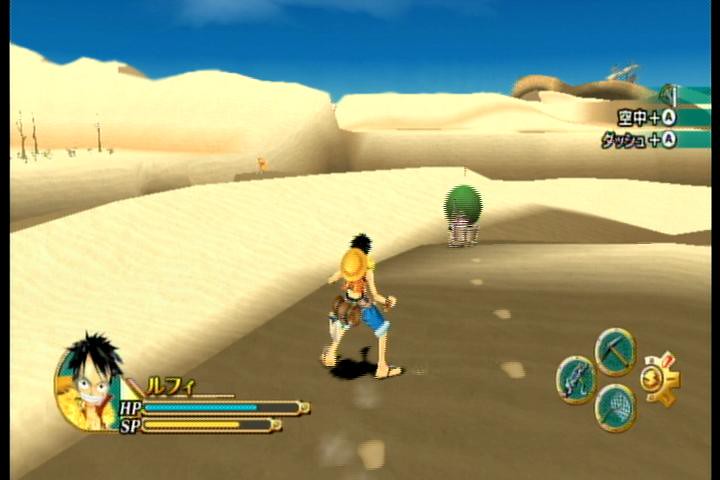Screenshot from a One Piece video game, featuring the character Luffy in a desert scene, likely from a PlayStation 2 era game. Luffy is clad in rolled-up jeans, flip-flops, and has his iconic straw hat slung behind his back. He stands with his back to the camera, revealing his black hair, while sand dunes stretch out into the horizon. Japanese text on the screen indicates this is the Japanese version of the game. The bottom right corner displays Luffy's HP and SP, accompanied by a vibrant image of Luffy looking intense. To the right, various items are visible, including a pickaxe and a net. In the distant background, faint structures and footprints add depth to the scene.